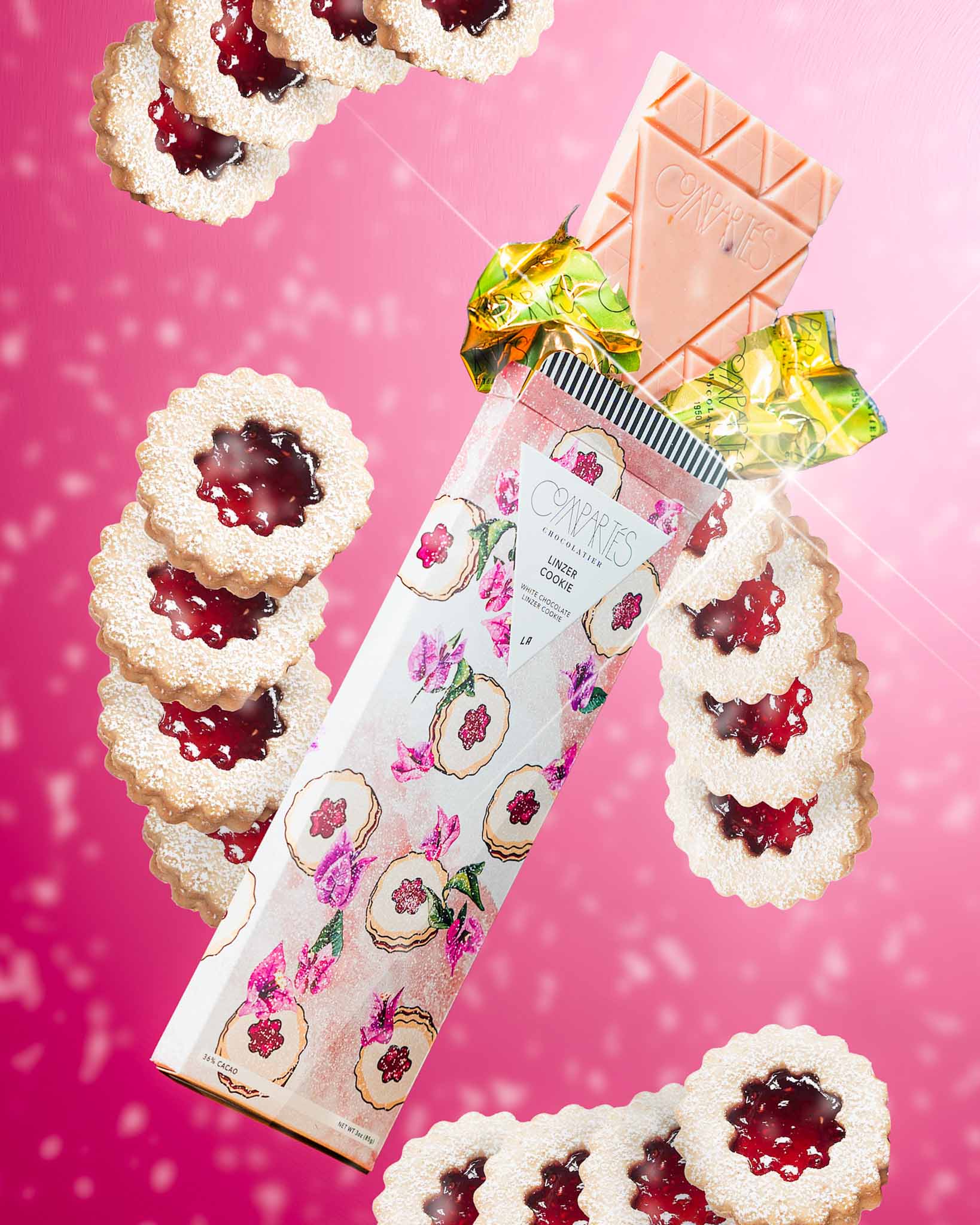In this vividly styled advertisement, a photograph showcases a luxurious candy bar and delectable cookies against a gradient pink backdrop. The background transitions from a darker pink in the lower left corner to a lighter pink in the upper right, speckled with tiny white dots. Central to the image is a half-unwrapped chocolate bar, revealing its golden foil interior and pink chocolate exterior. The bar itself is adorned with triangular divots and engraved branding, prominently displaying the white triangle logo reading "Compartes" and "Linzer Cookie" in slender black lettering.

Surrounding the chocolate bar, both within the wrapper design and scattered across the image, are elegant Linzer cookies. These cookies are circular with ruffled edges and a dusting of powdered sugar. Each cookie features a vibrant red jelly center, adding to the visual and presumably delicious appeal. The cohesive design, with cookies echoing the wrapper imagery, amplifies the upscale presentation aimed at enticing viewers.